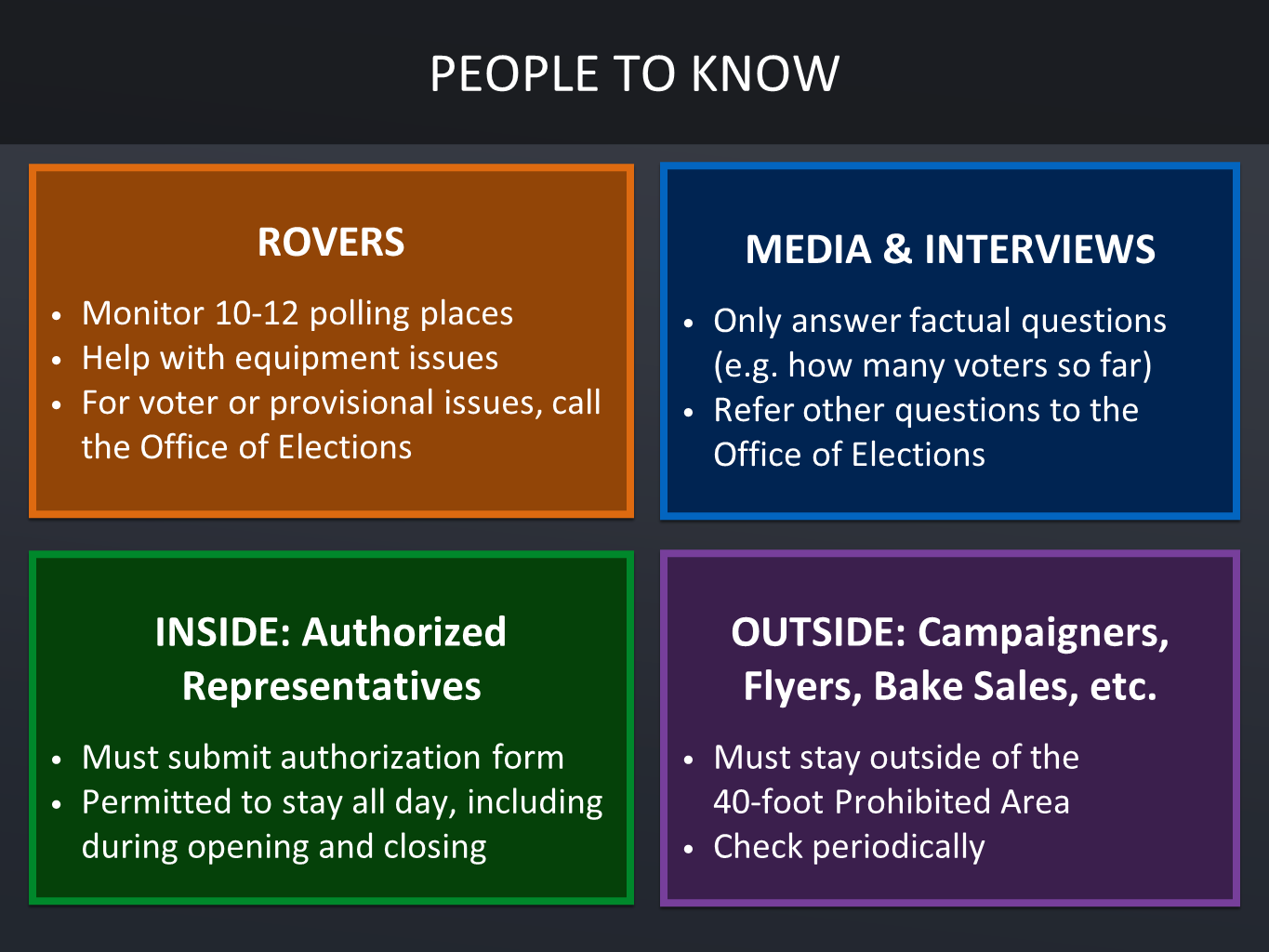The image depicts a motivational board or poster with a black background, featuring four distinct boxes surrounded by a gray border. At the top, prominently displayed in white and capitalized letters, it reads "PEOPLE TO KNOW." 

Beginning from the top left, the first box is orange-bordered and labeled "ROVERS" in white text. This box details roles such as monitoring 10 to 12 polling places, assisting with equipment issues, and addressing voter or provisional issues, with instructions to call the office of elections. 

To the right, the second box is blue and titled "MEDIA AND INTERVIEWS." It emphasizes only answering factual questions like voter turnout, while directing other inquiries to the office of elections.

On the bottom row, the left box is green with white text labeled "INSIDE AUTHORIZED REPRESENTATIVES." This section explains that representatives must submit an authorization form and are permitted to stay all day, including during opening and closing procedures.

The bottom right box is purple, titled "OUTSIDE CAMPAIGNERS, FLYERS, BAKE SALES, ETC." This box advises that such activities must remain outside the 40-foot prohibited area, with periodic checks to ensure compliance.

Each box categorizes specific roles and responsibilities, unified by the "PEOPLE TO KNOW" heading, and is visually distinguished by its color-coded borders.